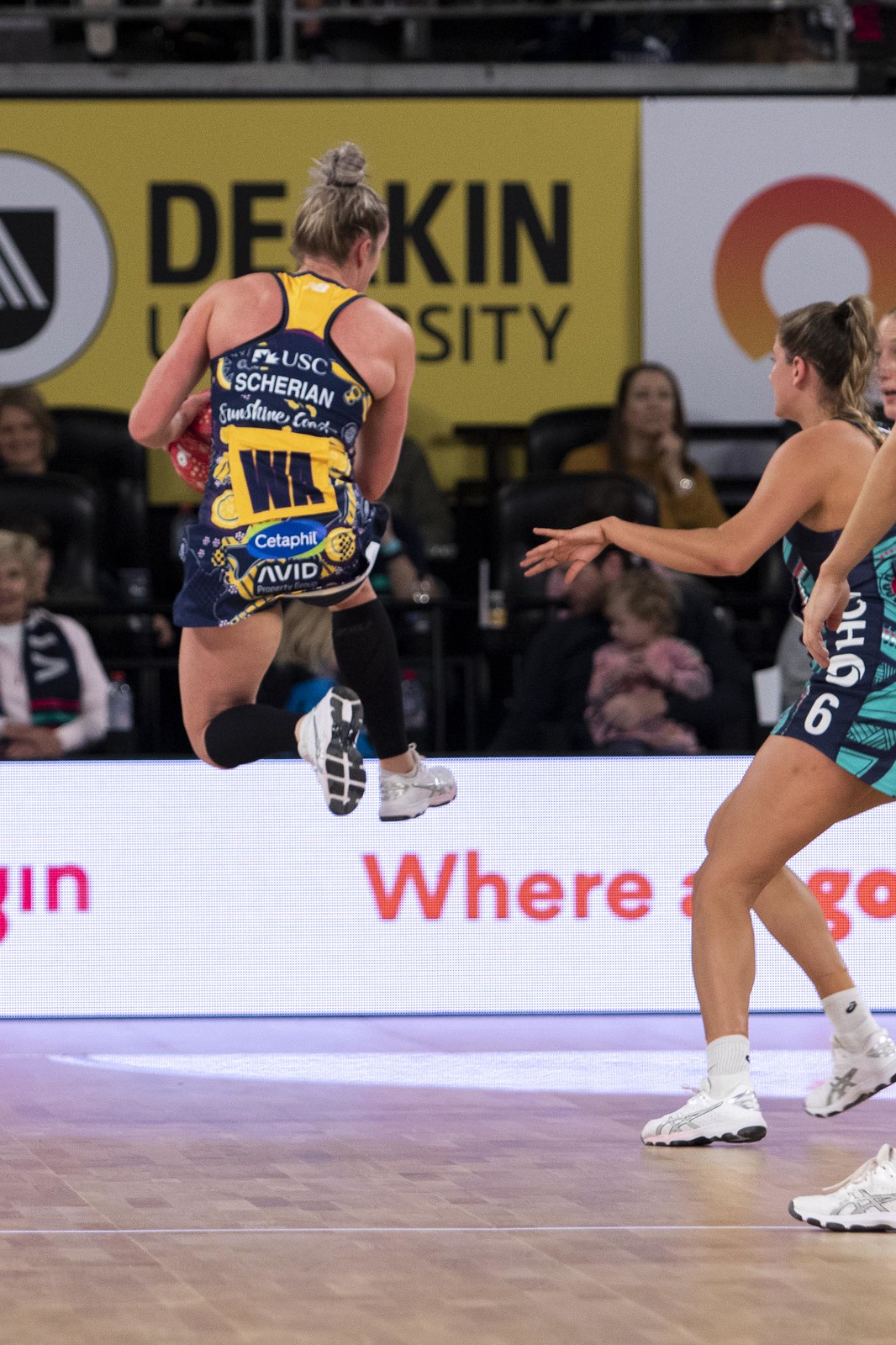This image captures an indoor athletic event, likely a volleyball match, featuring multiple female athletes. The scene is centered on a wooden floor, with the focus on a woman in a navy and yellow one-piece leotard, who is captured mid-air in an impressive jump. Her blonde hair is styled in a bun, and she wears high socks and white tennis shoes. She appears to be holding a ball under her left arm while extending her arms forward, suggesting an active play.

To the right of the airborne athlete, another woman is visible, dressed similarly in a one-piece uniform with advertisements, including names such as "USC, Sheeran, WA, Cetaphil, Avid." She has blonde hair tied back and stands on the ground with a determined stance, as if ready to engage with a play. We can also see part of another athlete's arm and leg at the edges of the photo.

In the background, a low white wall with red writing, possibly indicating team names or sponsors, separates the players from the spectators. Further behind, fans are seated, adding to the lively atmosphere of the sporting event. Various colors are present in the image, including shades of brown, white, red, dark blue, light blue, yellow, green, and navy, enhancing the dynamic and vibrant setting.